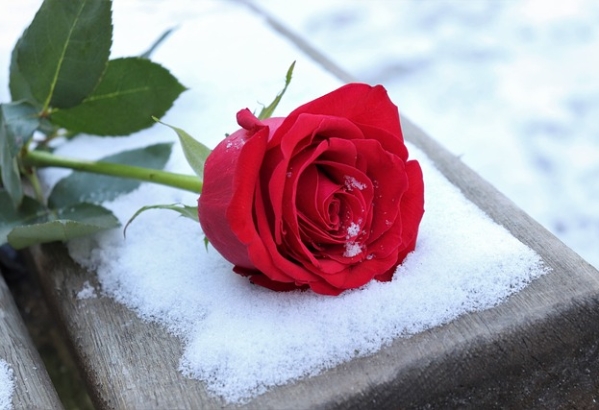A vibrant, deeply detailed red rose lies atop a weathered gray piece of wood, possibly a gravestone or a fence rail, covered with a thin, fresh layer of fluffy snow. The rose, with its velvety petals partially dusted with snowflakes, stands in stark contrast to the white wintery background. The stem and green leaves of the rose also show small traces of snow, emphasizing the season. The scene appears outdoors during the day, conveying deep symbolic significance, especially associated with love and remembrance in the afterlife. The vivid colors of the red petals and green foliage are accentuated against the serene white of the freshly fallen snow.